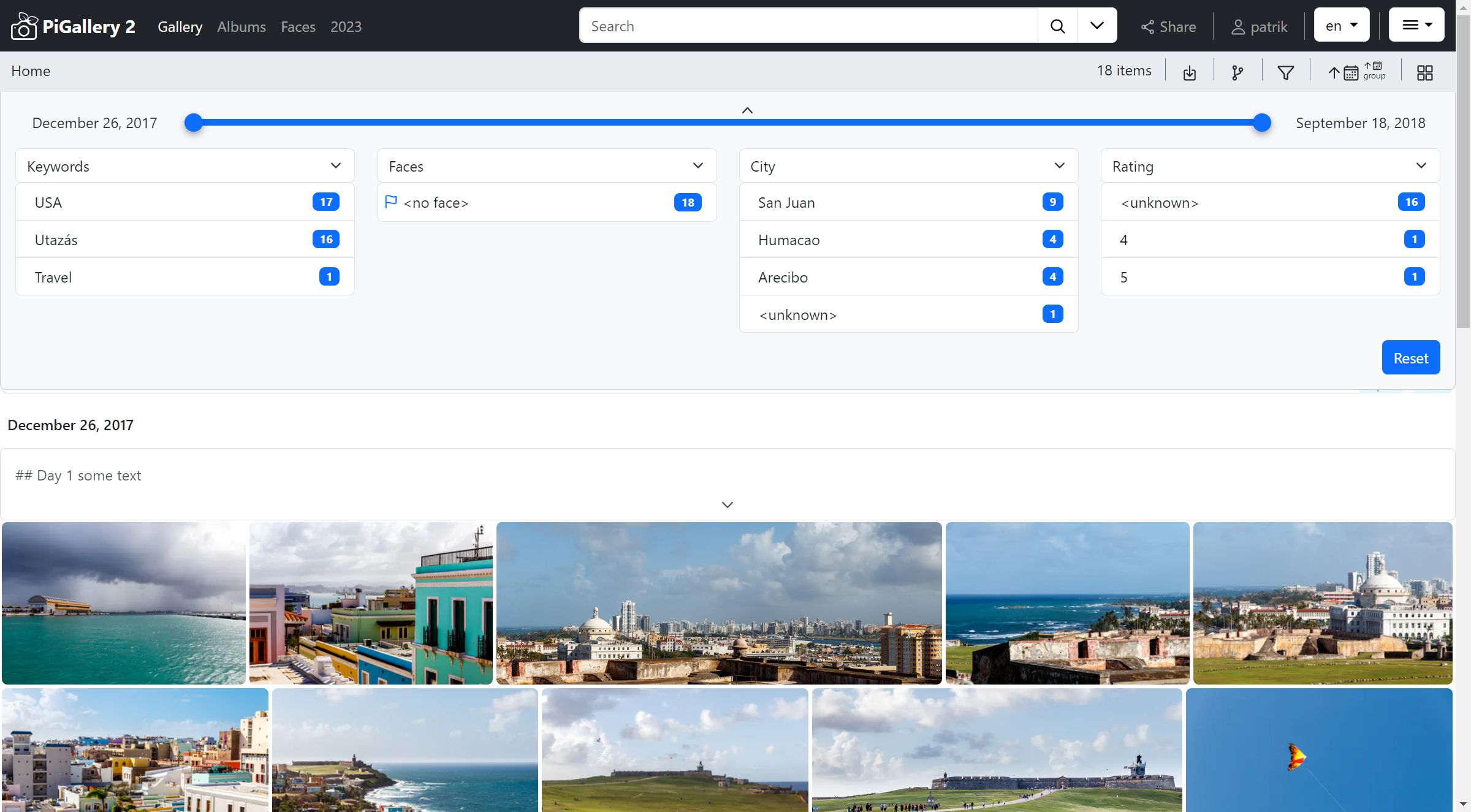The image caption provided describes a digital interface with various elements arranged in a structured format. Here's a cleaned-up and detailed version of the caption:

---

The top portion of the interface screen features a black bar with several elements. In the top left corner, the text "PI Gallery 2" is displayed in white. Adjacent to it is a small camera icon. Moving to the right, the words "Gallery Albums Faces 2023" are visible, accompanied by a white search bar. Further to the right, there is an option labeled "Share" followed by the text "Patrick" next to a small face icon. Additionally, two white drop-down boxes appear: one containing "n e n" and the other marked with lines, all set against the black background.

Below the black bar, the home section indicates "18 items" accompanied by several icons to the right. The dates "December 26, 2017" and "September 18, 2018" are displayed, separated by a blue bar. On the left side, under "Keywords," various keywords are listed including "USA," "Utah's," "US Travel," and corresponding blue numbers.

Further down, the "Faces" section shows "no face" with the number "18" next to it. Names such as "San Juan of Humacao," "RSC," "RSC Bow," and "Unknown" are displayed, each with associated numbers. In the "Rating" section, "Unknown" followed by "4/5" is noted, also with corresponding numbers, and there is a blue "Reset" button.

The section labeled "December 26, 2017" is titled "Day One," showcasing over 10 images depicting an outdoor cityscape. These images feature the ocean, cloudy skies, and various buildings, illustrating the scenic beauty of the location.

---

This detailed caption provides an organized and comprehensive description of the interface and its contents.